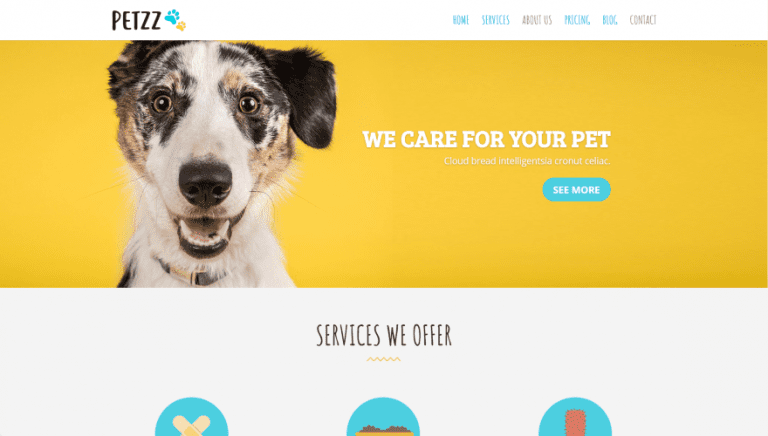The image depicts the PETZZ website, prominently featuring a logo consisting of a blue and yellow paw print. The site's navigation menu includes options such as Home, Services, About Us, Pricing, Blog, and Contact. Below the menu, there is a vibrant image of an excited dog with a white face adorned with black and brown spots, and an open mouth, looking eager.

The site's main text reads, "We care for your pet," accompanied by a blue "See More" button set against a bright yellow background. Below this section, there's another segment titled "Services We Offer," which features three icons on blue backgrounds. The first icon, in beige colors, forms an X shape. The second icon shows dark colors at the top with lighter brown below, resembling food. The third icon, in red, appears to depict a sponge, possibly for cleaning. The "Services We Offer" section is displayed on a gray background with the title in black text.